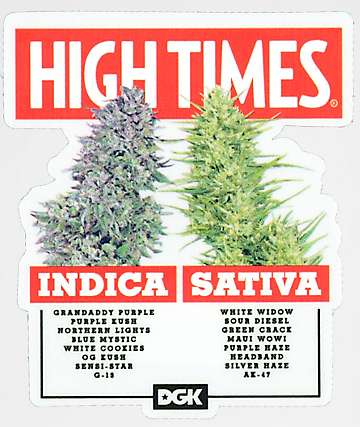This image from High Times magazine is an advertisement for various strains of marijuana. The background is all white, featuring a bold red rectangular banner at the top with the words "High Times" in capital white letters. To the left, there is an image of a dense, purplish-green Indica marijuana plant, labeled "Indica" in large white letters on a red background. Below this, in dark font, are the strain names: Granddaddy Purple, Purple Kush, Northern Lights, Blue Mystic, White Cookies, OG Kush, and Sensi Star G13. On the right, a vibrant green Sativa plant is shown, labeled "Sativa" in the same white letters on a red background. Below this plant are the strain names: White Widow, Sour Diesel, Green Seabuck, Maui Waui, Purple Haze, Headband, Silver Haze, and AK-47. At the bottom of the image is a black rectangle with the white letters "DGK," with a star inside the "D." This advertisement highlights various popular marijuana strains, categorized into Indica and Sativa.